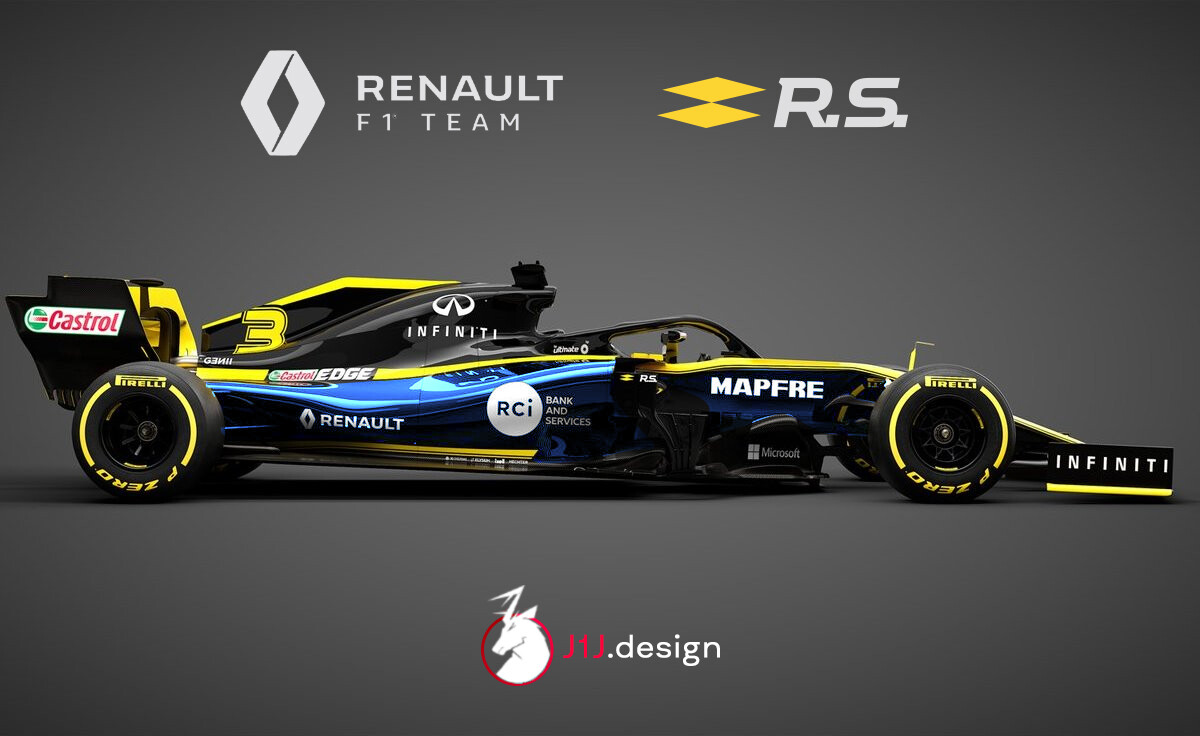The image showcases a Renault F1 team race car, predominantly black with striking yellow lines running along its body and detailed blue accents on the side. Positioned against a gray and black background, the car features a prominent Renault F1 Team logo at the top. Adjacent to this logo are two yellow triangles with the initials "R.S" in white lettering. The race car displays various sponsor logos, including Infiniti on the front and Castrol as a sticker on the rear wing. Additionally, there are logos for MAPFRE, RCI Bank & Services, Microsoft, and Pirelli P-Zero tires highlighted with yellow edges. The car, marked with the number three, sits above a logo featuring a deer inside a red circle, labeled "J1J.design."